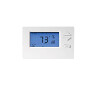This image depicts a very small section of a thermostat or control panel for an HVAC system. The device features a white plastic cover that surrounds a blue LED screen situated on the left side of the panel. The screen displays black characters, most notably the number "73". The screen is cast in shadow at the top, and a small, indiscernible black squiggle appears on the upper right side of the display, accompanied by some black lines beneath it. To the right of the LED screen are two physical buttons shaped like triangles – one pointing up and the other pointing down, indicating their function to increase or decrease temperature settings. These buttons are prominently protruding, designed for tactile interaction. Additional minor artifacts or pixelation appear in the bottom left corner of the image, making it hard to discern specific details.